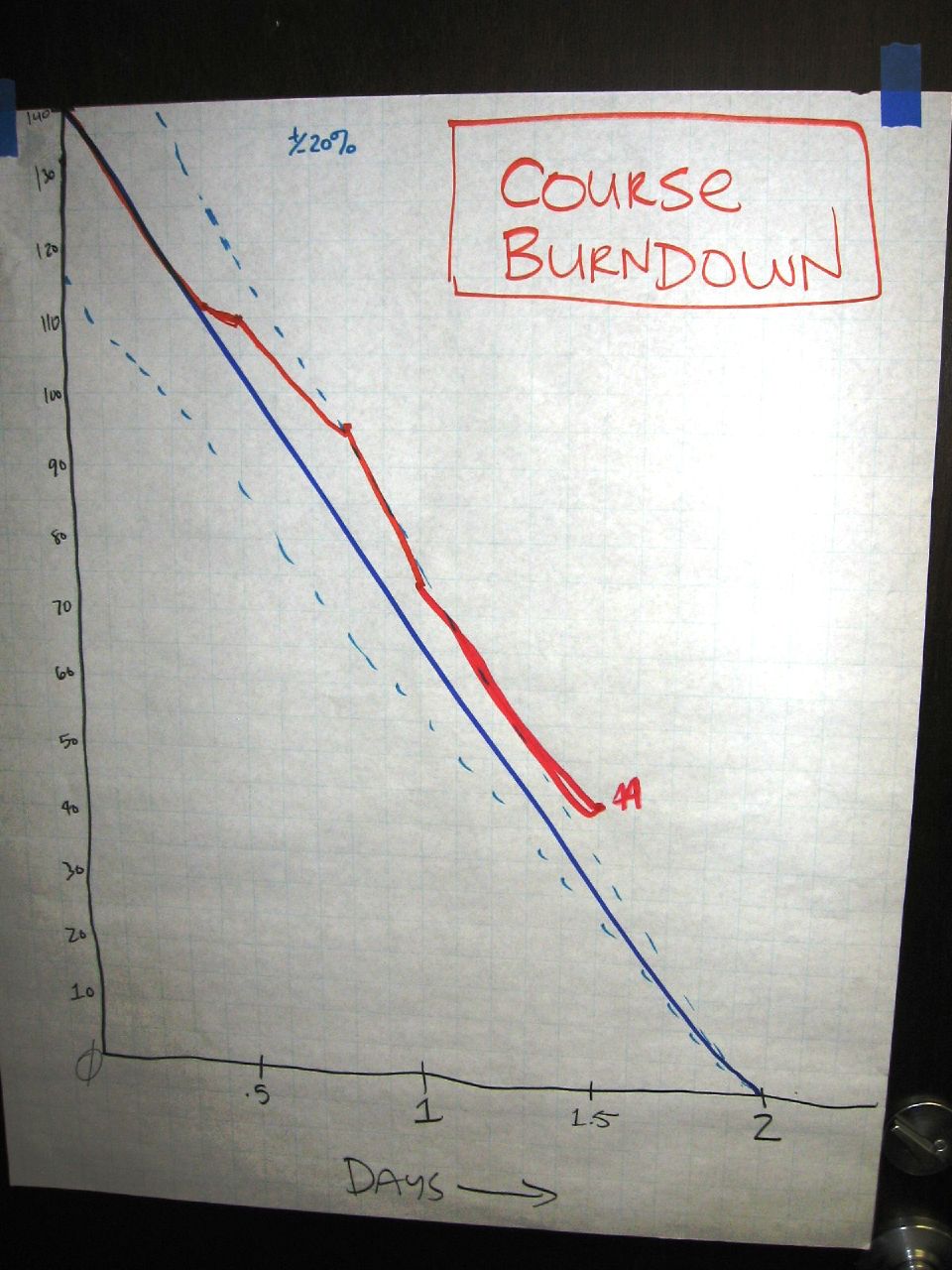This photograph showcases a detailed line graph drawn on graph paper, which is affixed to a door with blue tape at the top right corner. The background of the graph paper features blue lines running across and down. The main content of the graph includes a black X-axis labeled "Days" with an arrow pointing to the right, ranging from 0 to 2 in intervals of 0.5, and a black Y-axis numbered in increments of 10 from 0 at the bottom to 140 at the top. 

Two primary lines are prominent in the graph: a blue line that starts at 140 on the Y-axis and slopes diagonally downwards to meet the X-axis at 2, and a red line that begins parallel to the blue line but curves off around the X-axis point of 1.5, ending just past it. Additionally, there are two dotted blue lines on either side of the graph, tapering towards the blue line as they approach the X-axis at the value of 2.

In the top center of the image, "+/- 20%" is written in blue. Above this is a red rectangular box containing the title "Course Burndown" in red text. The bottom right corner of the photograph reveals part of the door with a visible doorknob and lock, indicating the image was likely taken in a casual or home office setting.